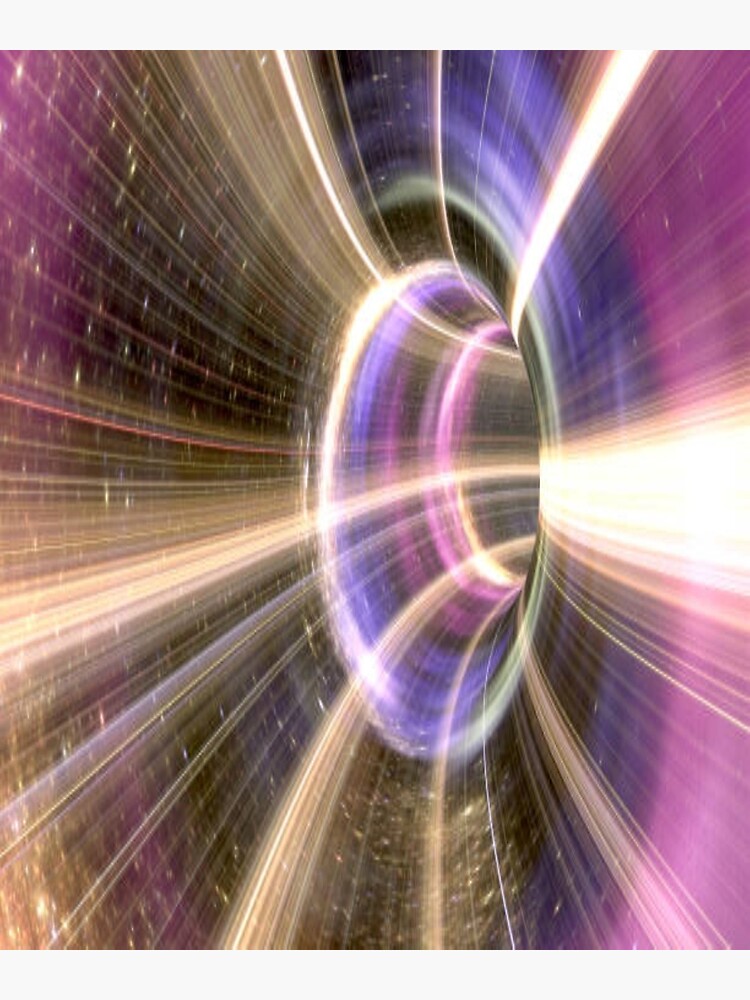This highly detailed and visually striking artwork, likely computer-generated, illustrates an elongated black hole or wormhole in space. The viewer is presented with an illusion of swiftly moving into or through the cosmic phenomenon, encapsulated by vivid ribbons and swishes of light that diverge into the distance. Dominated by shades of purple, blue, white, reds, and violet, the scene is set against a dark backdrop peppered with stars. The light flows into the black hole, creating an almost tunnel-like pathway that curves, evoking a sense of rapid motion similar to that experienced on a roller coaster. The bright, multidimensional lights and textured layering enhance the depiction of a surreal, otherworldly journey through space, offering a hauntingly beautiful perspective of a black hole.